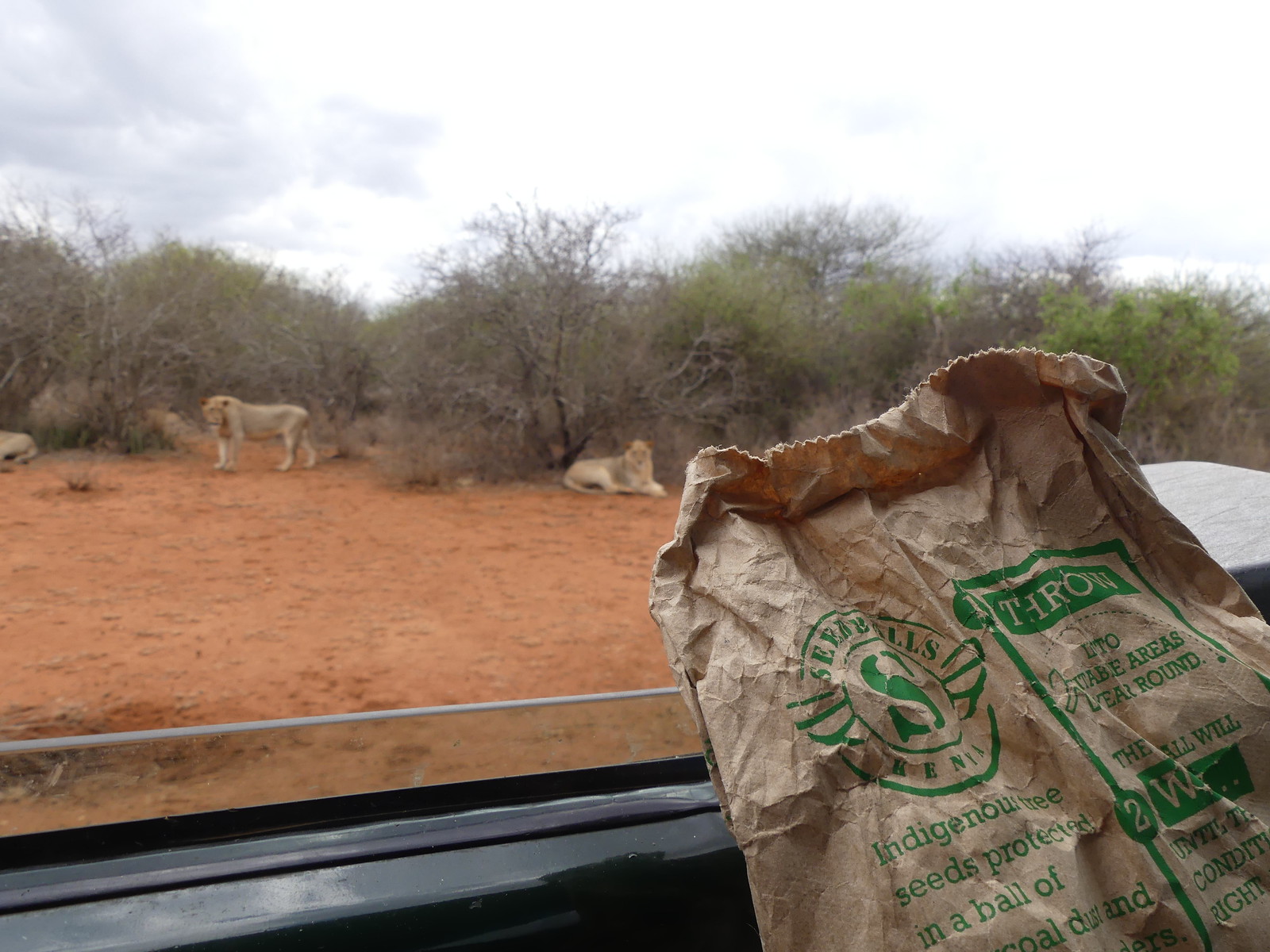In the image taken from inside a vehicle, possibly in a safari park in Africa, a brown paper bag with green writing about indigenous tree seeds leans against the window, partially obscuring a rearview mirror. Outside, the landscape features orangish-brown dirt, shrubs, and small, sparsely leafed trees. On the left side of the scene, two tawny lions rest near the brush. One lion stands, gazing leftward with its mane visible behind its head. Beside it, a second lion lies down, legs outstretched and tail curled, looking directly at the vehicle. The sky above is overcast and hazy. No people are visible in the photograph.